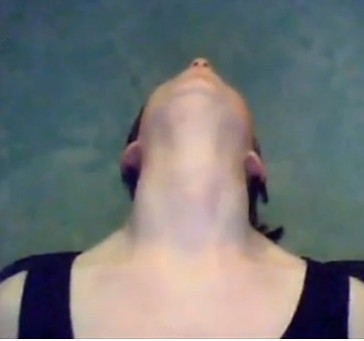This is a color square photograph featuring a person, likely a white male, holding their head tilted all the way back. The background is mottled in shades of light gray, green, and blue, giving an impression of a wall in poor quality. The person has brown hair that falls to their shoulders and is wearing a navy blue or black tank top, which exposes their thick neck, shoulders, and upper chest. Their pale skin has pink undertones, especially noticeable around the neck and ears. Only the person's nostrils, lips, the underside of their nose, and earlobes are visible. The image appears somewhat filtered, adding to the ambiguity of whether it is a photograph or an oil painting.